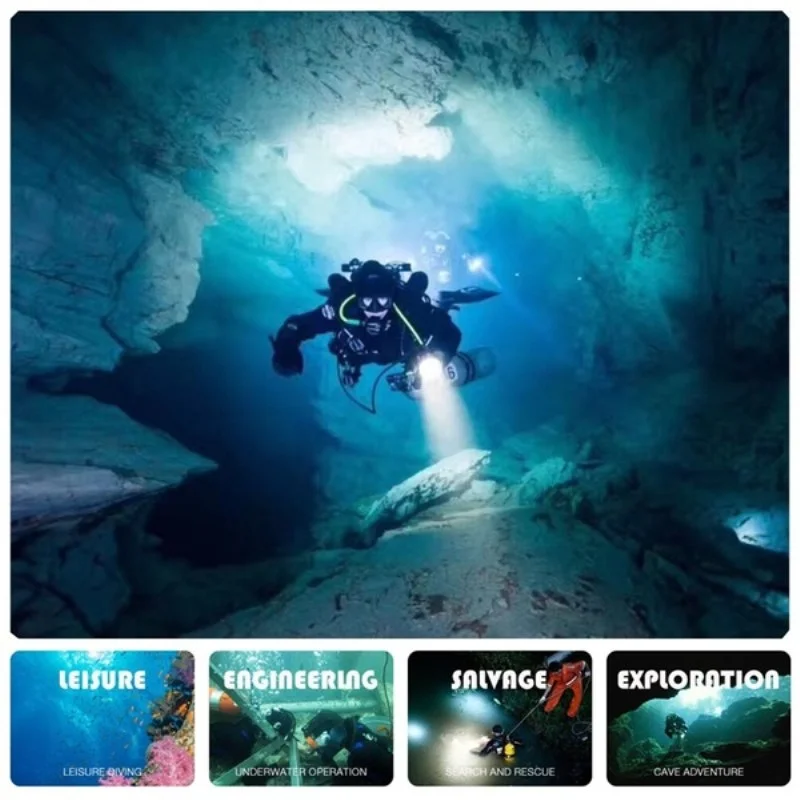The image is a detailed advertisement for a diving company that specializes in a range of underwater activities, including Leisure, Engineering, Salvage, and Exploration. In the main photograph, a scuba diver is seen exploring an underwater cave, holding a flashlight in their left hand and fully equipped with scuba gear, including a mask and flippers. The water around them is a striking blue, and beneath them lies a tunnel-like system of underground rocks. Behind the main diver, another person with a flashlight can be seen, further illuminating the cave. The lower portion of the advertisement features four distinct images labeled: "Leisure" with an image of blue water and coral, "Engineering" showing a diver working on underwater equipment, "Salvage" depicting a search and rescue operation with a man looking through the water, and "Exploration," which highlights a diver navigating an intricate underwater cave system. The overall color scheme is dominated by blues and aquamarine, with the divers' suits primarily black, accented by green hoses and white flashlight beams. This vividly showcases the adventurous and specialized services offered by the diving company.